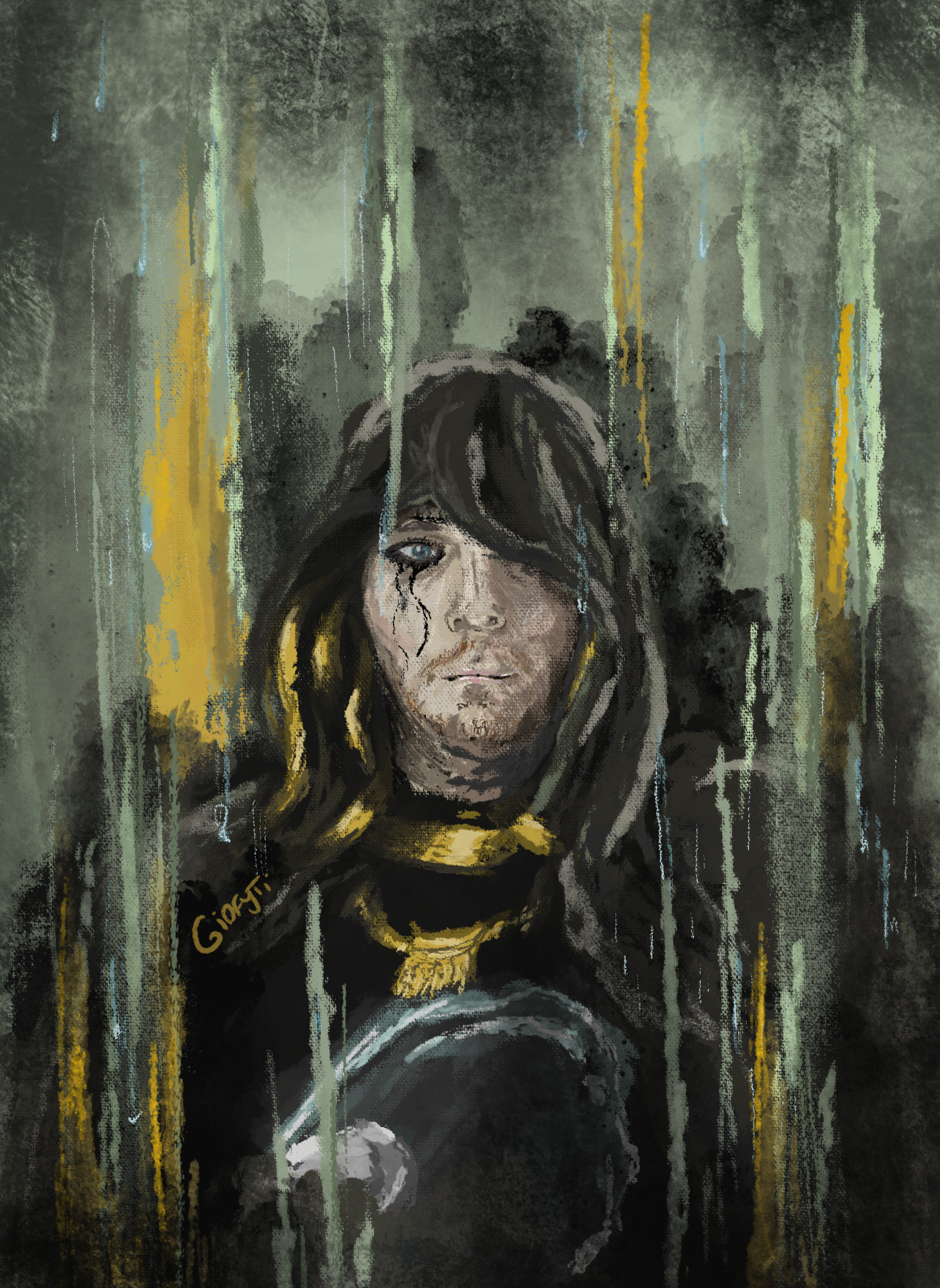The painting portrays a solemn figure, centered and wearing a dark, medieval-style cloak with an intricate blend of black, yellow, and green hues against a splotchy backdrop reminiscent of a stormy sky. The background, with its dynamic streaks of black and hints of yellow and green, feels almost as if the paint is cascading down like rain. The man in the image has long hair obscuring his right eye, with only his piercing blue left eye visible, adorned with what appears to be a smudge of black mascara running down his cheek, suggesting either rain or tears. He has a light beard, along with a brown goatee and mustache. His mouth is closed, and he gazes intently into the distance. The cloak he wears is black with yellow designs, possibly a robe with gold accents around the neck and inside, including an emblem on his chest and a golden tie. There is an inscription on his right shoulder, which appears to be the artist's signature, potentially reading "Giorgio." The overall ambiance of the painting is dark and somber, enriched with intricate details and a sense of mystery.